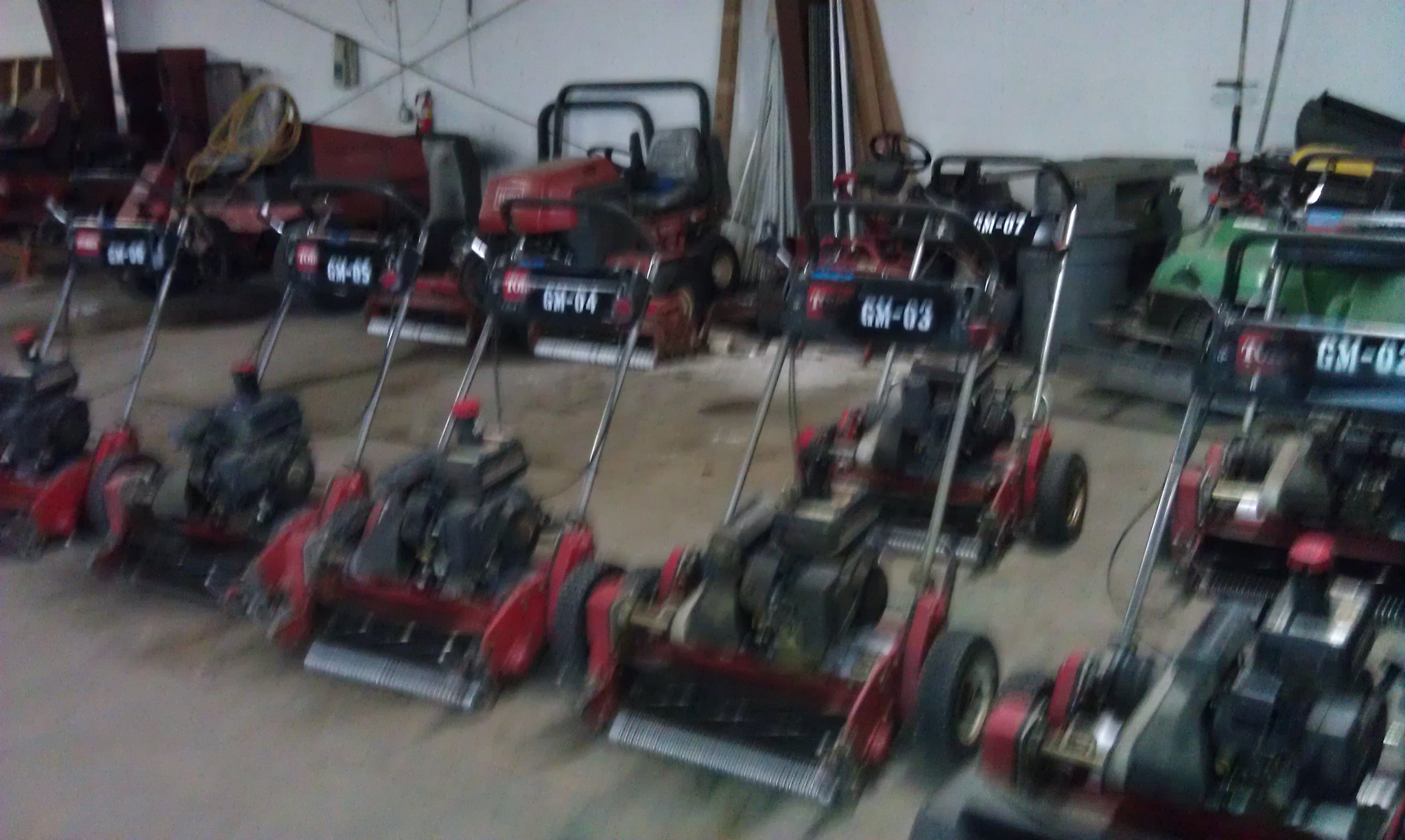The image captures an indoor storage space with a concrete floor, featuring approximately 11 lawnmowers neatly lined up in rows. The front row consists of red Toro lawnmowers, all identical in size, shape, model, and color, characterized by black safety handles and seats. The handles have labels such as GM03, GM04, and GM05, written in white letters on a red background. These machines have two wheels each, with blades in the front and an engine or motor on top. In the back row, there are predominantly red lawnmowers accompanied by one or two green lawnmowers. The storage area, which resembles a garage, also contains a trash can next to one of the green machines and some hanging fabric that appears to be a car cover. The white walls accent the industrial nature of the setting, showcasing a variety of yard equipment.